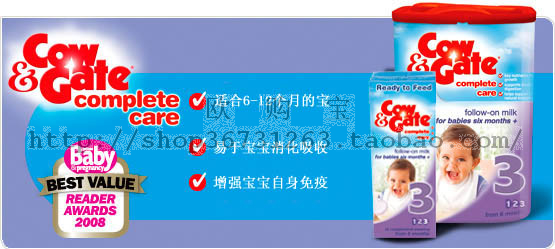The advertisement features a bluish-purple, periwinkle-toned background with prominent text and visuals. In the top left corner, the red text reads "Cow and Gate Complete Care," and below it is a logo for the "Baby Pregnancy Best Value Reader Awards 2008." Next to the logo, three white checkmarks are present, each accompanied by Chinese characters to their right. On the right side of the image, two products are displayed. The larger product is a package of baby formula with a red lid and the label "Cow and Gate Complete Care" in red. Below it, in blue text, it states "Follow on Milk for Babies 6 Months Plus," accompanied by a picture of a smiling baby wearing a white bib and a large number "3." Adjacent to this is a smaller, similar package labeled "Ready to Feed," also featuring a baby's face.